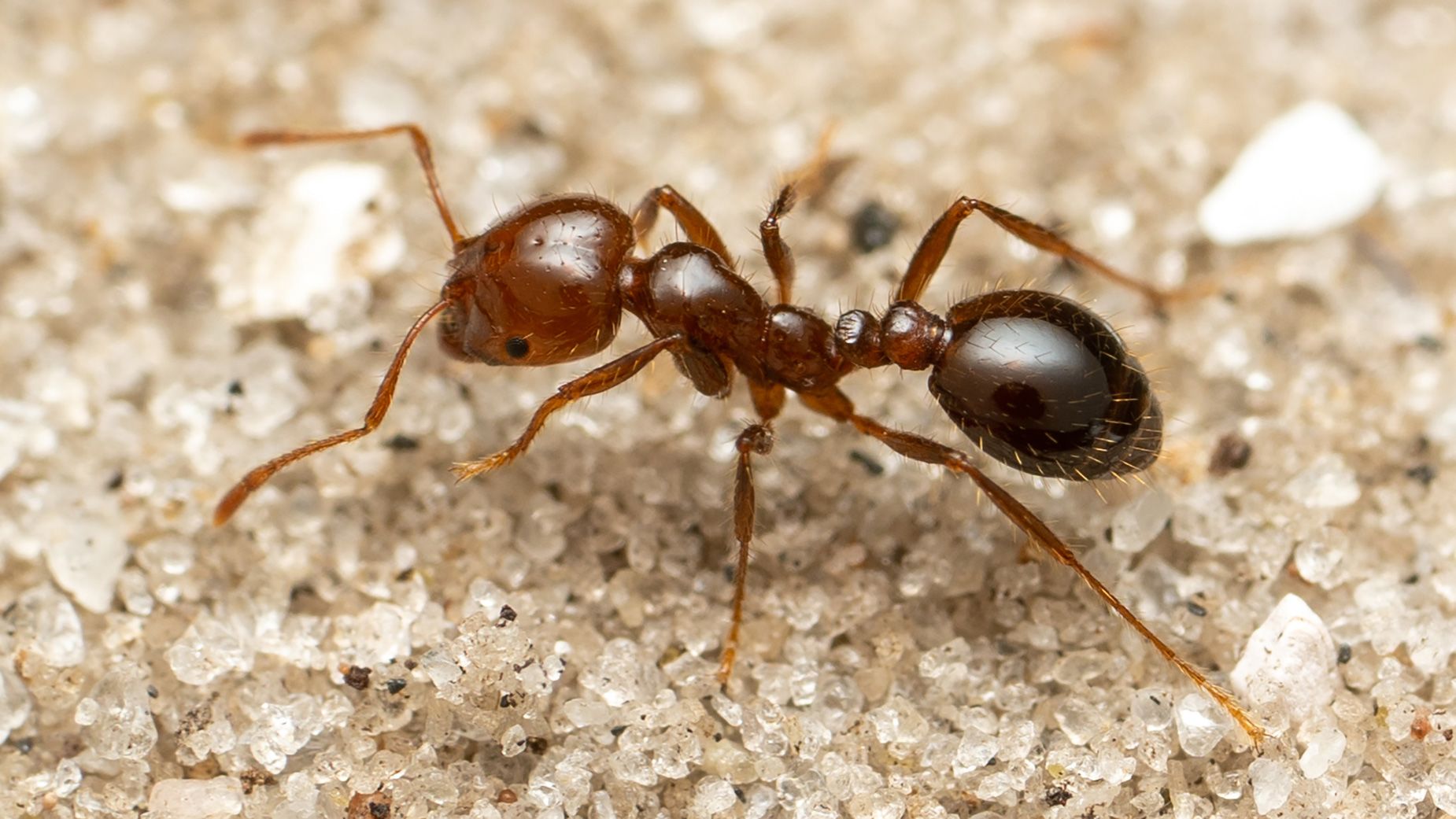This image is a color photograph of a close-up of a brownish, dark brown ant, magnified to highlight its detailed features. The ant, with its characteristic six legs and two long antennae, is positioned on a surface that resembles a bed of clear, crystal-like pebbles, possibly sand or rock salt. The ant's body parts, including a large head, thorax, and a darker abdomen with a prominent bubble-like shape at the tail, are clearly visible. It's covered in fine, tiny hairs, especially noticeable on its thorax and legs. One of its eyes, located on the left side of its head, stands out in this highly detailed image. The lighting suggests that the photograph was taken indoors, adding to the clarity and sharpness of the intricate details.